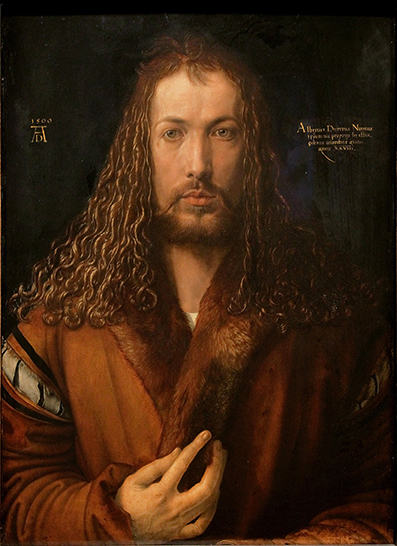This detailed oil painting portrays a man, likely of royal or notable status, suggested by his ornate attire and regal posture. The subject, possibly a prince or a king, has long, partly curly hair that extends past his shoulders, a feature accompanied by a dark red, slightly curly beard and a matching goatee-mustache combination. His hair and facial hair are tinged with shades of brown and dark red, contributing to his distinguished appearance.

He is adorned in a coat with a prominent, luxurious fur collar that is brownish-red in hue, accented by white sections on the shoulders. The background of the painting is dark, providing a stark contrast that highlights the subject's features and attire. 

To the right of his face, there is text that barely discernible spells out possibly the name "Albert," although the full text cannot be determined. There’s also mention of a date, with speculations ranging from 1500 to 1800, written in a stylized manner. On the left side, additional illegible text seems to further identify the man or the artist. Notably, the painting exudes the stylistic elements of a Renaissance artwork, reflective of its detailed craftsmanship and period feel.